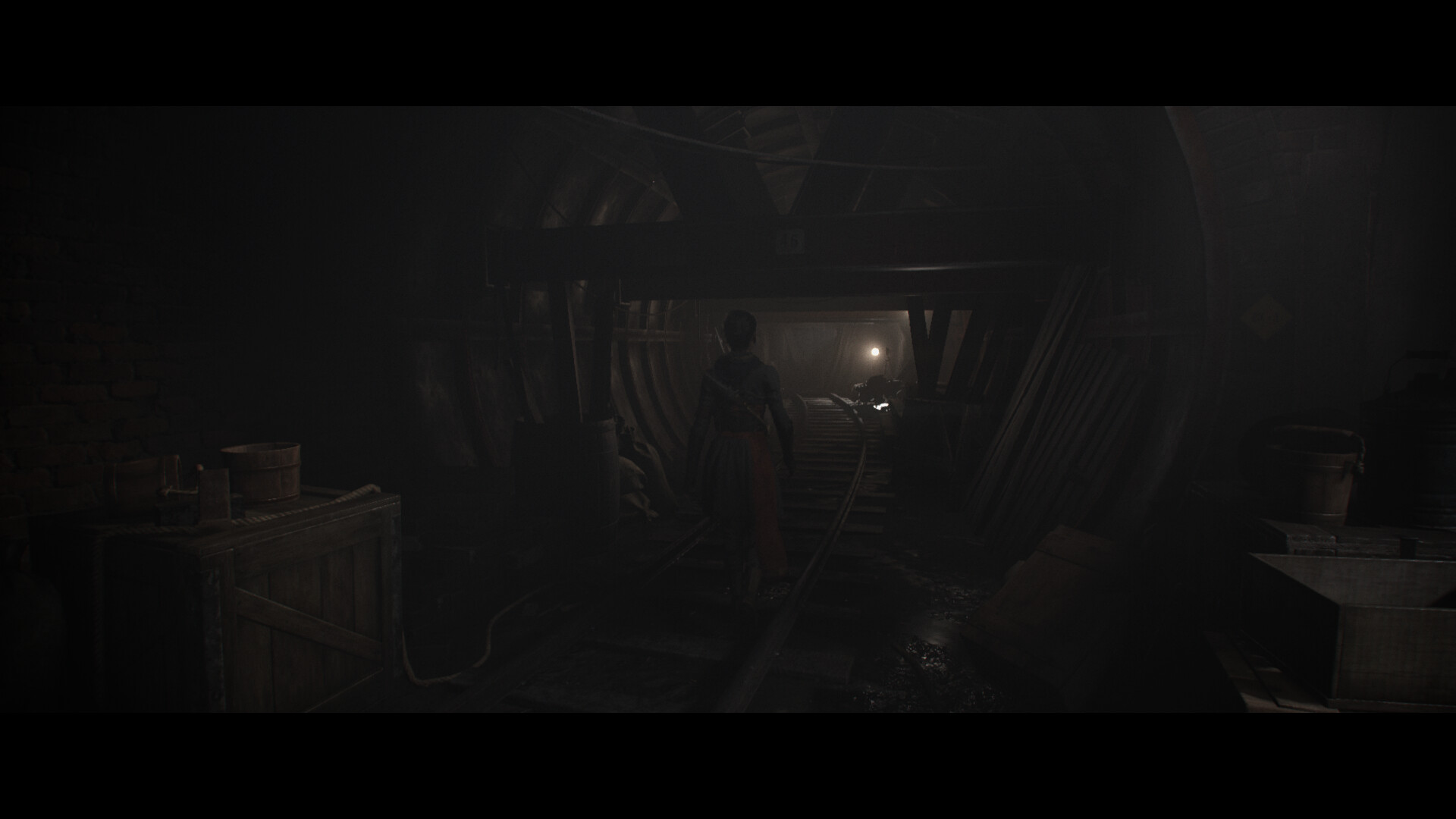The image depicts a dark and shadowy underground tunnel, resembling a mine shaft or an old railroad tunnel, with wooden pillars and beams supporting its structure. In the foreground, a wooden crate is visible. The scene is shrouded in darkness, requiring careful observation to discern details. At the center, a faint light source at the end of the tunnel illuminates the silhouette of a person, walking away from the viewer towards the light. The individual wears a strap across their chest, but their features and identity remain indistinguishable in the gloom. The person is framed against the old wooden supports of the tunnel, creating an eerie and mysterious atmosphere.